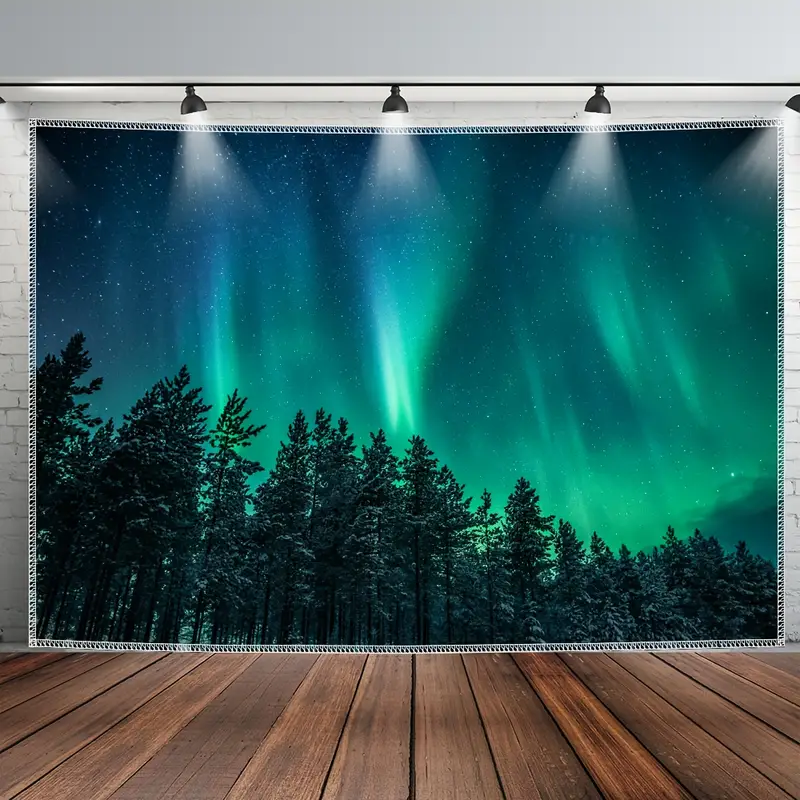The image depicts a realistic, square-shaped photograph set in an interior space. The bottom part of the image features dark, rustic mahogany hardwood floor planks running vertically towards the center. The top portion reveals a light gray wall resembling a cement surface designed to look like white-painted brick. Horizontally aligned along the top of the image is a black track bar adorned with five black light fixtures that cast white light downwards.

Central to the image is a large hanging piece, which could be a screen, a painting, or a cloth, showcasing a vivid and enchanting night sky. The night sky is predominantly black and dark blue, highlighted with streaks of green and blue, possibly representing the Northern Lights. Along the base of this centerpiece are silhouettes of dark pine trees, indicating a magical forest night scene. The sky in the image has a gradient effect, blending from dark blues to lighter greens, evoking a serene yet mystical atmosphere of nature illuminated by the Northern Lights. The overall setup aims to capture the natural beauty of a starry, luminous night against the backdrop of a forest. The centerpiece, bordered by a subtle white mesh, dominates the visual space and is accentuated by the lighting fixtures above.